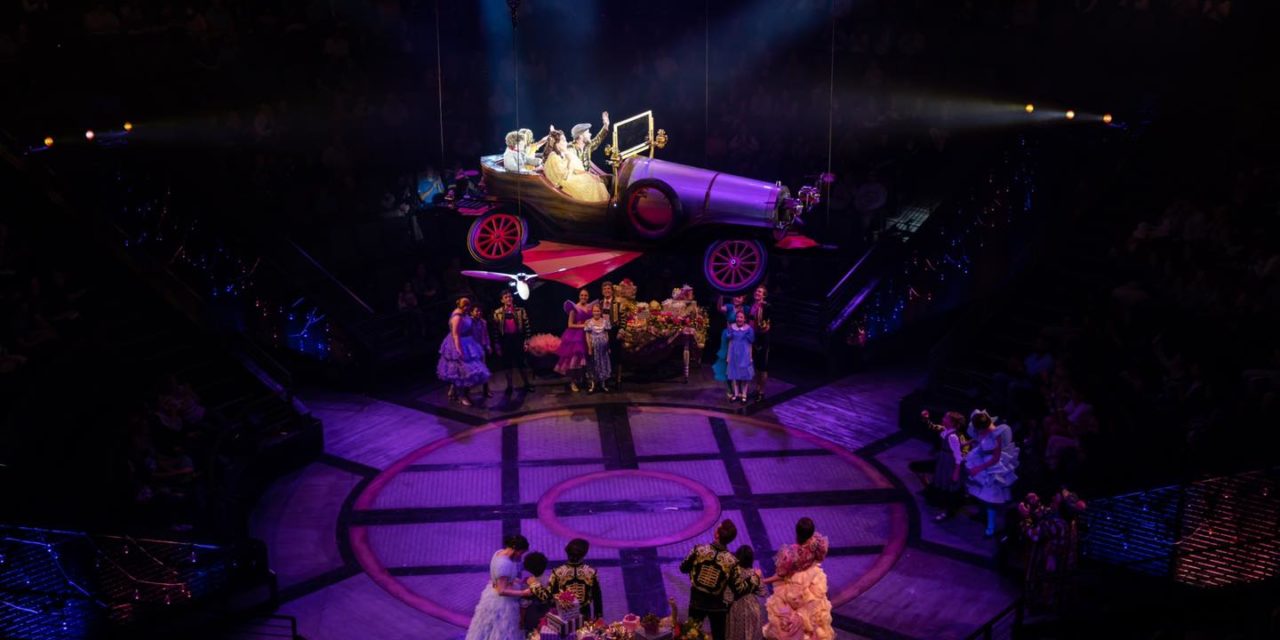The photograph captures a vibrant, theatrical stage set during a musical performance. The stage is round with four illuminated walkways leading up to it, and the background is dark, punctuated by small, yellow stage lights. At the center of the stage hovers a large, vintage automobile, resembling an early 20th-century model with a purple front and red wheels. This vehicle, suspended mid-air, houses four individuals who are waving to the crowd below. The crowd on stage, dressed in period costumes including flowy gowns and outfits reminiscent of royalty or bullfighters, gazes up at the floating vehicle. The stage itself is decorated with vibrant colors—purples, pinks, and blues—highlighted by a pink-outlined circle and a pattern of black lines crisscrossing the floor. The dynamic scene is filled with energy and historical flair, as both the costumes and the props transport the audience to a bygone era.